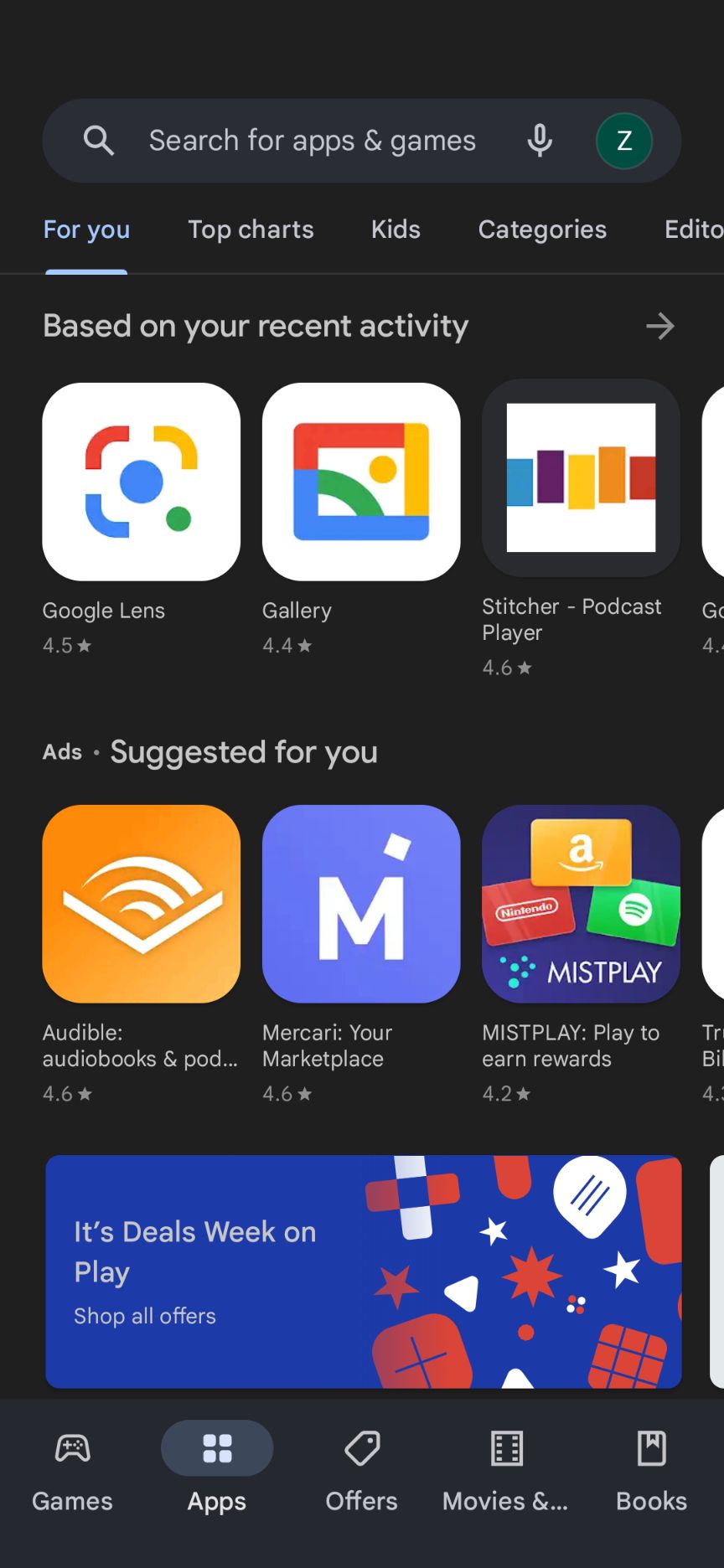This image appears to be a screenshot from a smartphone displaying the Google Play Store. The screen features a search bar at the top, indicating that the user is searching for games and apps. Below the search bar is a section titled "Suggested for you," which recommends various apps and games to the user. 

The background is predominantly dark, providing contrast to the colorful app icons and text. In the "Suggested for you" section, the top row includes app icons for Google Lens, Gallery, and the Stitcher Podcast Player. Below that row, there are more recommended apps: Audible (for audiobooks), Mercari (a marketplace app), and Misplay (an app that appears to offer rewards for playing games). 

At the bottom of the screen, a banner announces "Deal Week on Play," suggesting that there are special offers or discounts available on the Google Play Store. Further down, there are icons representing different categories such as games, apps, movies and TV shows, and books. Each category icon links to its respective section where users can explore more options in that genre.

Additionally, under the "Misplay" app, there are recognizable brand icons such as Amazon and potentially Nintendo, indicating associated offers or content. 

Overall, the screenshot gives a detailed view of the Google Play Store's interface, highlighting personalized app recommendations and promotional deals.